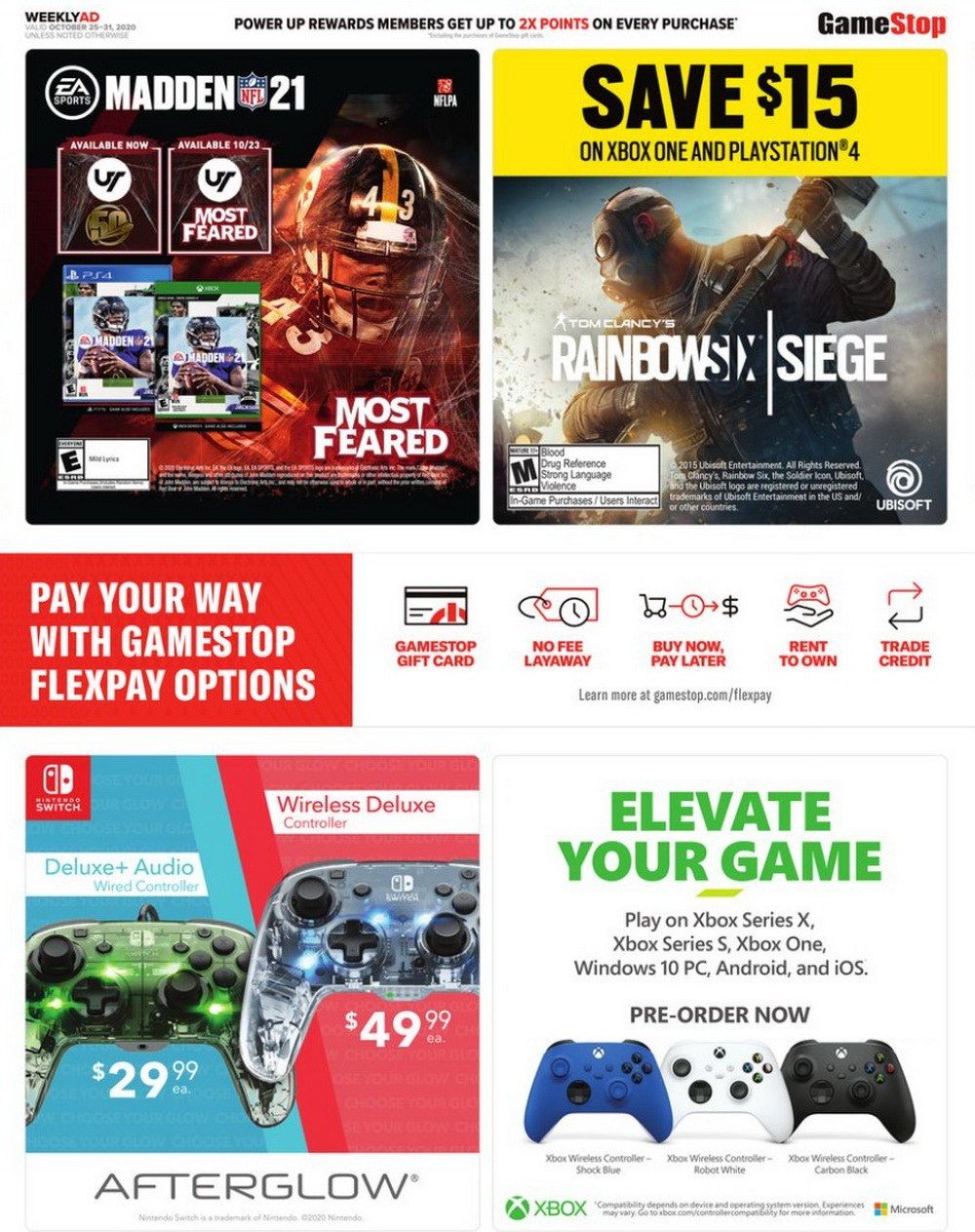---

**Power Up Rewards Event (October 24th - 30th, 2020)**

This week, Power Up Rewards members have the opportunity to earn up to 2 test points and win various prizes, including games and merchandise. Featured prominently is Madden 21, which showcases a football player donning a helmet with dynamic lines emitting from him. The game, released on October 23rd, 2020, is highlighted for its wide appeal, particularly in Texas.

Madden 21 is currently priced at $15 for Xbox One, PlayStation 4, and Sega Saturn. Another notable game in the spotlight is Tom Clancy's Rainbow Six Siege, known for its intense themes such as blood, drug use, warfare, strong language, and violence. The promotion also mentions the option to purchase exclusive t-shirts via the app.

Promotional section details include:

- **Top right:** UPSOFT logo
- **Bottom left:** Red Square logo and GameStop FlexPay options, including gift cards, no-fee layaway, and buy now, pay later. 

Visual elements feature a person extending their hand with a controller above them. The scene is colored with a red tone and arrows pointing right and up-left to indicate various directions.

Specific product highlights:
- **Nintendo Switch Wired Controller:** Deluxe Plus Audio at $29.98
- **Wireless Deluxe Controller:** Priced at $49.99 with a highlighted version named "Afterglow."

Taglines such as "Elevate Your Game" emphasize the enhancement of the gaming experience. The promotion encourages playing on platforms like Xbox Series X, Xbox One, Windows 10 PC, Android, iOS, and with routers.

The visual scheme consists of blue, white, and black elements, with an Xbox logo prominently located. Microsoft's logo appears on the right side, adding brand authority to the event.

---